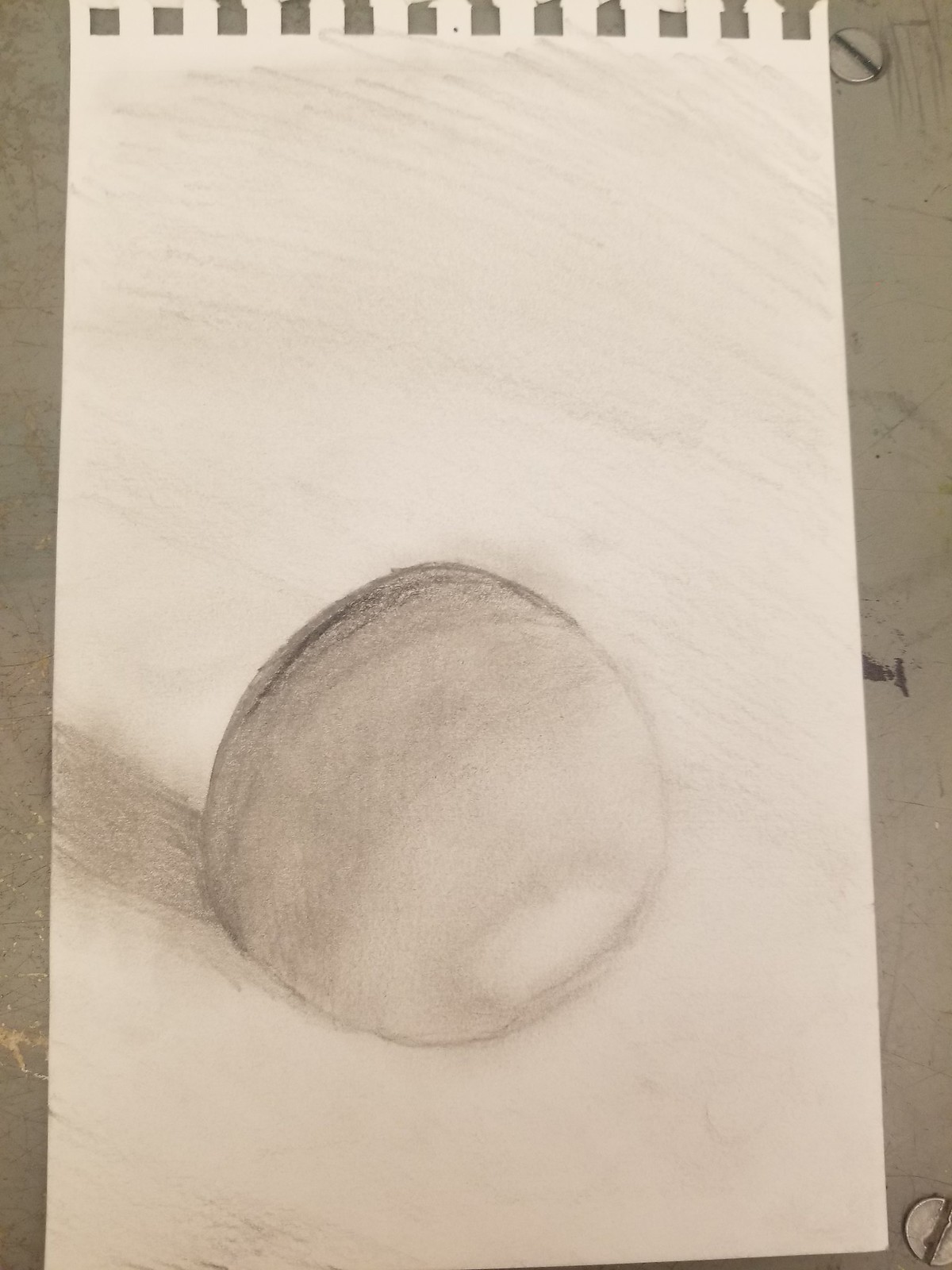The image depicts a pencil sketch on a piece of sketch paper that has been torn out of a sketchbook, evident from the square holes along the top. The sketch is of an imperfect, lopsided sphere, resembling a cross between an egg and a golf ball. The sphere is shaded darker at the back, with the front lighter, and includes smudgy lines on the left indicating a shadow cast behind and to the left of the object. This drawing is done on sepia-toned paper, which is placed on a matching sepia-toned table. The background of the sketch paper features faint horizontal streaks, with visible bolts or screws at the top right and bottom right corners.